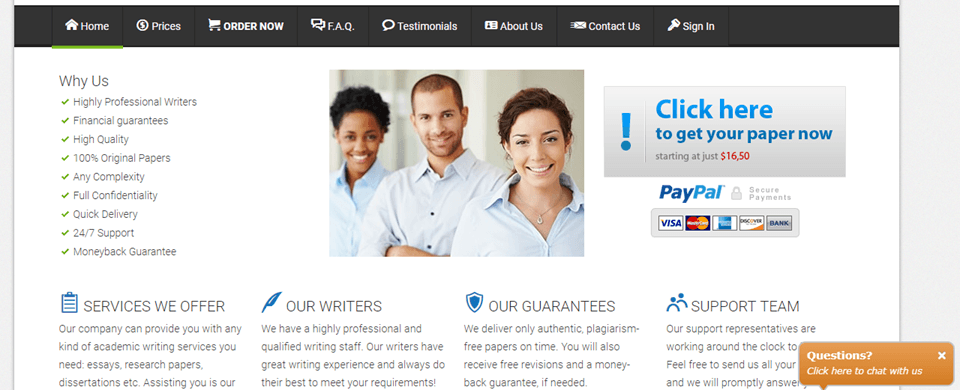**Detailed Caption:**

The promotional image features a group of three diverse individuals, centrally positioned and exuding a welcoming and professional demeanor. In the middle stands an African American woman with short black hair, donning a blue shirt, with a broad, inviting smile. To her left, a Caucasian male with a close-cropped haircut, also clad in a blue shirt, has his arms folded confidently, matching her bright smile. In front of them both is a Caucasian woman with sleek black hair, also wearing a blue shirt and a stunning diamond pendant necklace. She shares the same cheerful expression, completing this trio of approachable professionals.

The background is a pristine white, suggesting a clean and modern environment, possibly an office building. Above the group, there is a navigation bar set against a blackboard-like background displaying various options such as "Home," "Prices," "Order Now," "FAQs," "Testimonials," "About Us," "Contact," and a "Sign In" button. A conspicuous link encourages users to "Get your paper now starting at just $6.50," indicating affordability.

The image further outlines multiple payment options, including PayPal, Visa, MasterCard, American Express, Discover, and bank cards, emphasizing convenience and security. Key features of the services are highlighted, such as the promise of highly professional writers, high-quality and 100% original papers, handling high complexity tasks, maintaining full confidentiality, quick delivery, 24/7 support, and a money-back guarantee.

These services cater to various academic writing needs, including essays, research papers, and dissertations. The assurance of authenticity, with no plagiarism and free revisions upon request, further enhances the reliability of the service. Additionally, the support team’s round-the-clock availability encourages users to seek assistance at any time. A bright orange chat button is prominently placed in the lower right-hand corner, inviting users to initiate a conversation for any issues or inquiries.

The overall presentation is clean and inviting, making the webpage appear professional and user-friendly, poised to meet diverse academic writing needs.